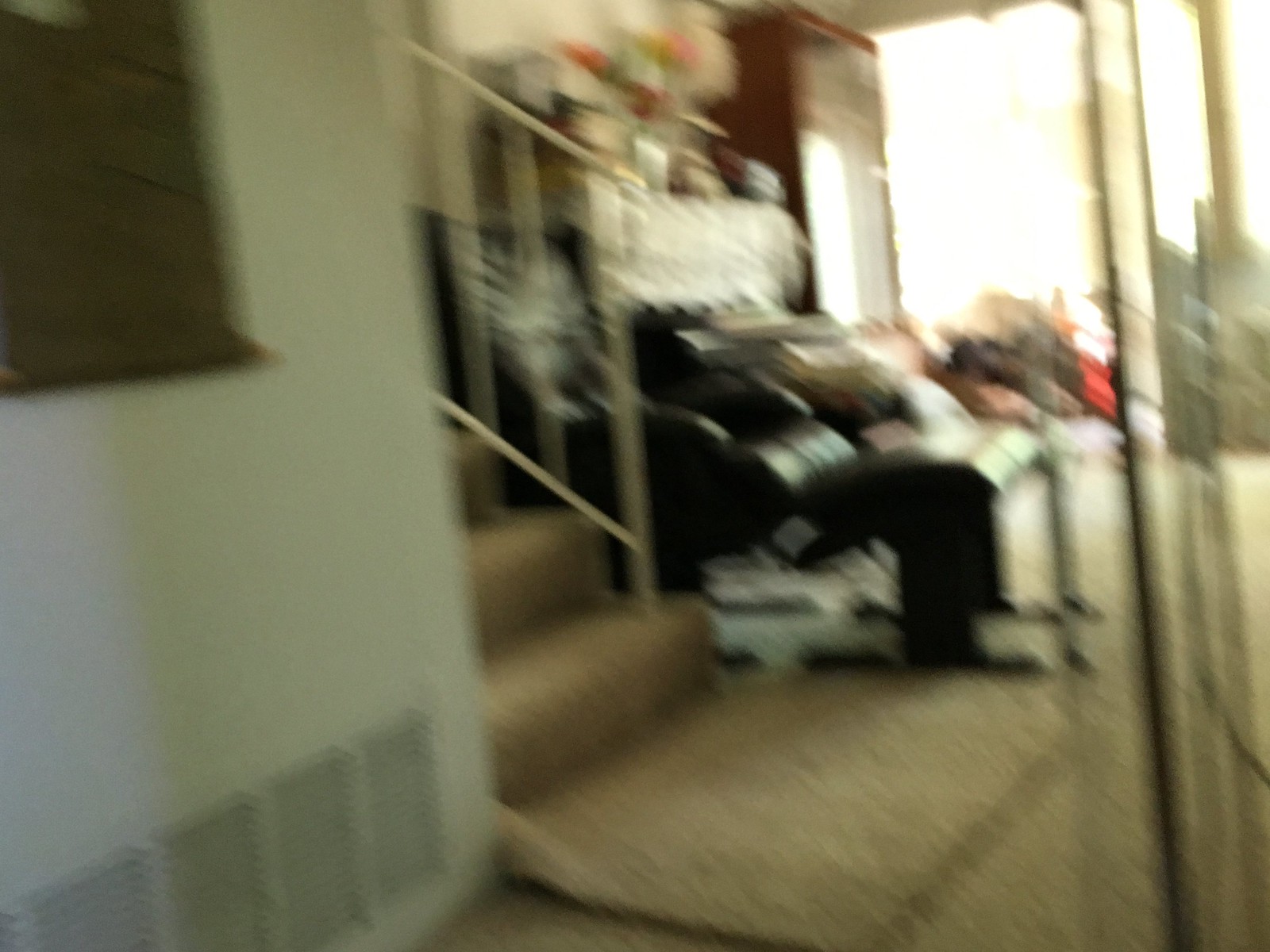The image, though blurred, offers a glimpse into the interior of a house, focusing on several key areas. In the bottom right corner, there are four evenly spaced vents. The top right corner features a painting hanging on the wall, adding an artistic touch to the space. Centered in the image is a staircase, characterized by sleek silver railings and brown carpeting, providing a transition between the different levels of the house. 

To the top right of the image, a glass window is visible, through which natural sunlight filters, casting a warm yellow glow into the room. On the right-hand side, a semi-translucent, transparent structure, possibly a door, accentuates the modern design of the interior. Centrally positioned in the image is a table, accompanied by a seat where one can comfortably put their feet up, suggesting a relaxed, inviting atmosphere. The gym and living room areas are subtly hinted at, contributing to the multifunctional nature of this household space.